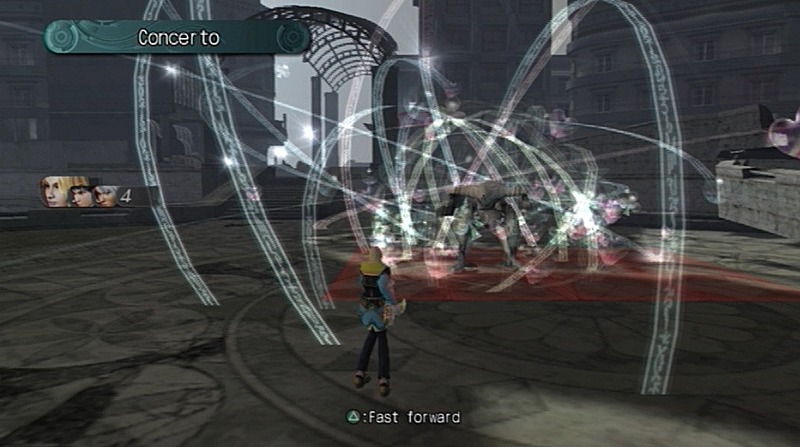This detailed image appears to be a screenshot from a vintage PlayStation game, likely from the years 2007 to 2009. The scene is set in a dark, possibly nighttime, environment that evokes a futuristic or cyberpunk aesthetic. At the top left corner, there's a blue-teal banner with the word "Concerto" in white letters, possibly indicating the level or title of the scene. Below that, a digital display shows a "Cancer 2" heading along with an indicator of characters, displaying the numbers "4" and "3."

The center of the image features a figure with their back to the viewer, dressed in black armor, a black vest, blue shirt, black pants, and black shoes, and could possibly be wearing a hat. The figure stands amidst a flurry of radiant, white lines and sparkles that resemble ribbons or light trails, adding to the intense action of the scene. These light effects emanate from the character and arc gracefully around the scene, contributing to the sense of motion and combat.

At the bottom of the image, a familiar PlayStation HUD element shows a green triangle labeled "Fast Forward." The area beneath this character seems to be a red carpeted floor, suggesting a significant battleground or stage. Surrounding this central figure are various elements including a drum set or band equipment to the front, spotlit areas, and in the upper right corner, a white tablecloth on a table. 

The left side of the image displays pictures of faces with a digital number "4" next to them, possibly indicating team members or characters in play. The right side reveals stacks of concrete and distant, shadowy buildings, enhancing the environment's gritty, industrial feel. Overall, the image combines elements of a fighting scene with musical and performance motifs, set against a moody, immersive backdrop.